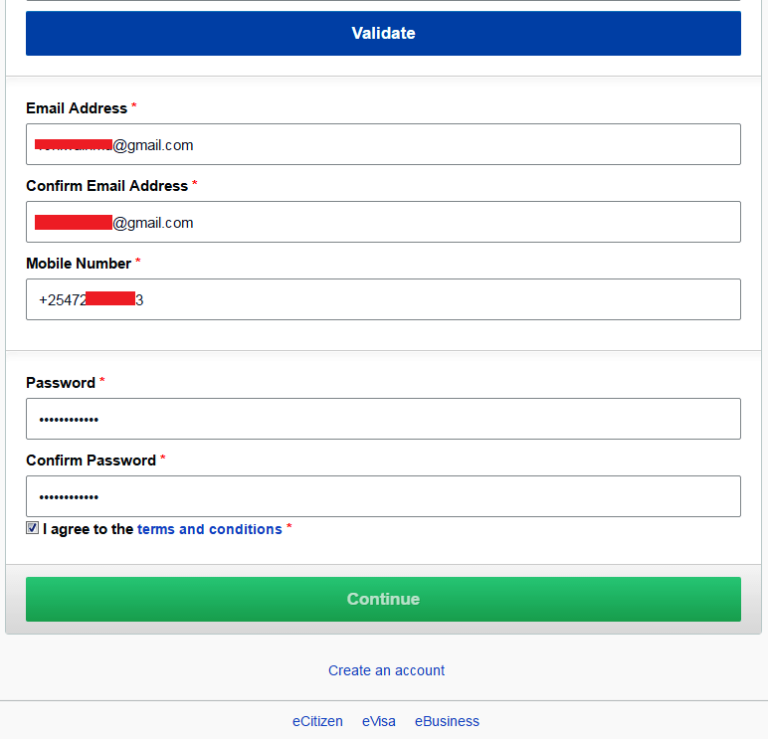The image displays a user registration form with a white background. At the top of the form, there is a thin black line. Directly below this line is a large blue button that spans the width of the form, labeled "Validate" in white text. Further down, there is another thin black line. Below this, the form asks for the user's "Email Address," marked with a red asterisk indicating a required field. The input field shows an email partly redacted with a red overlay, revealing only "@gmail.com".

Next is a "Confirm Address" field, also marked with a red asterisk. The content is identical to the "Email Address" field, with the text partially redacted in the same way. Following this is a "Mobile Number" input field, indicated as mandatory with a red asterisk. The field displays a partially redacted number starting with "+25472" and ending with a "3".

Below another horizontal line, the form requires a "Password" entry, signified by a red asterisk, with the input field displaying obscured characters (dots). The subsequent field, "Confirm Password," equally marked with a red asterisk, also shows obscured characters in its data field.

Near the bottom of the form, there is a square checkbox followed by the statement "I agree to the Terms and Conditions," where "Terms and Conditions" is highlighted in blue, with a red asterisk indicating this consent is required. Finally, at the bottom of the form, there is a green button labeled "Continue".